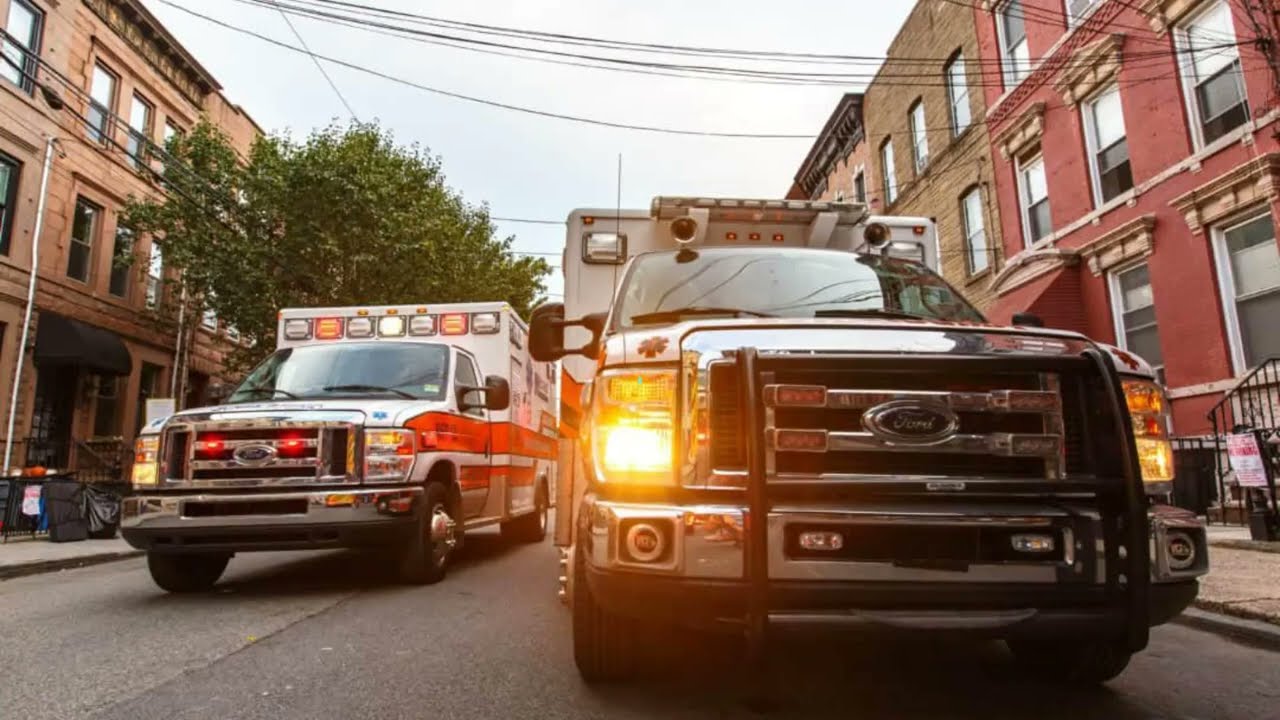The photograph captures a straight-on view of two Ford ambulances driving down a street in an urban setting, likely New York City. The ambulance on the right is closest, prominently displaying its grill, headlights, and the blue Ford emblem. This vehicle's headlights are on, and two red lights flash on either side of the emblem. The other ambulance, slightly farther away to the left, shows a red stripe along its side and also has its lights on. Both ambulances are moving towards the viewer, occupying the entire street. Flanking the scene are three-story brick apartment buildings with black canopies over the entrances and a sidewalk running alongside. The scene includes additional elements like trash cans, and in the background, a clear sky and a large tree can be seen. Colors in the image range from the white and red of the ambulances to the various hues of the buildings and other surroundings.